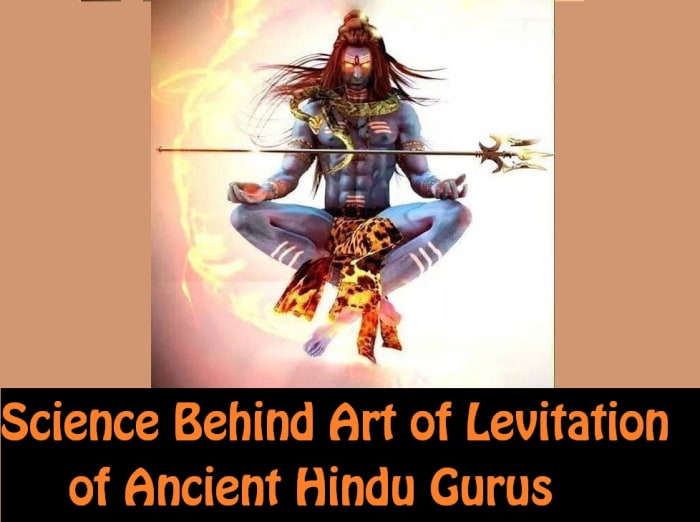In the center of the image, a detailed color illustration depicts a muscular blue-skinned man performing a magical levitation trick. His legs are crossed in a lotus meditation pose and he is floating mid-air, gazing directly at the viewer with glowing orange eyes. His long brown hair flows around him, adding to the mystical atmosphere, enhanced by swirling magical mist and flames in the background.

The man is adorned with intricate face makeup and white markings on his eyes, chest, belly button, and calves. He holds his hands on his knees, palms facing up, with a golden trident, or spear with three points, levitating above each palm. A snake, coiled around his neck, adds to his enigmatic appearance. The only garment he wears is a loincloth with a wildcat or cheetah pattern.

The scene is bordered by two uniform pale tan vertical rectangles on both sides, extending from a black rectangle at the bottom of the image. This black rectangle contains the text "Science Behind Art of Levitation of Ancient Hindu Gurus" in orange. This text is also repeated within the image itself, seamlessly merging ancient mysticism with a scientific context.